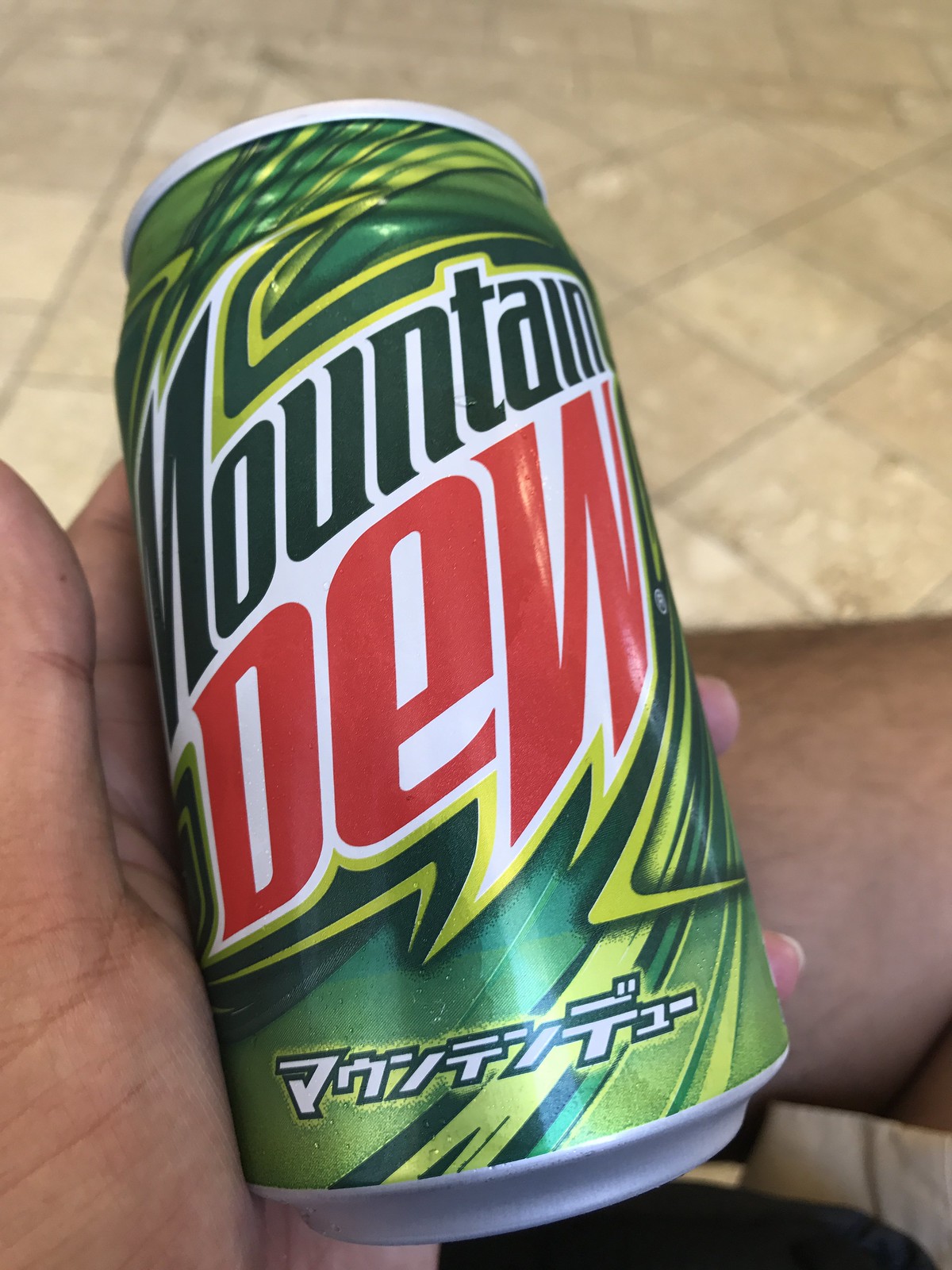The image is a close-up color photograph of a Mountain Dew can, prominently held by a person's left hand. The can, which dominates the photo, features the familiar Mountain Dew logo with "Mountain" in green and "Dew" in red, set against a vibrant green background with patterns resembling leaves in various shades of green. Notably, there is Japanese katakana text displayed at the bottom of the can, indicating it might have been purchased in Japan. The can has a silver bottom and top. The person's hand, with medium dark skin, wraps around the can, with two fingers visible on its edge. The person is wearing beige shorts and a dark shirt, and appears to be sitting on a white tiled floor with their legs crossed. The background includes a blurred area of beige, diamond-shaped tiles. The overall scene suggests a casual setting where someone is showcasing the can.